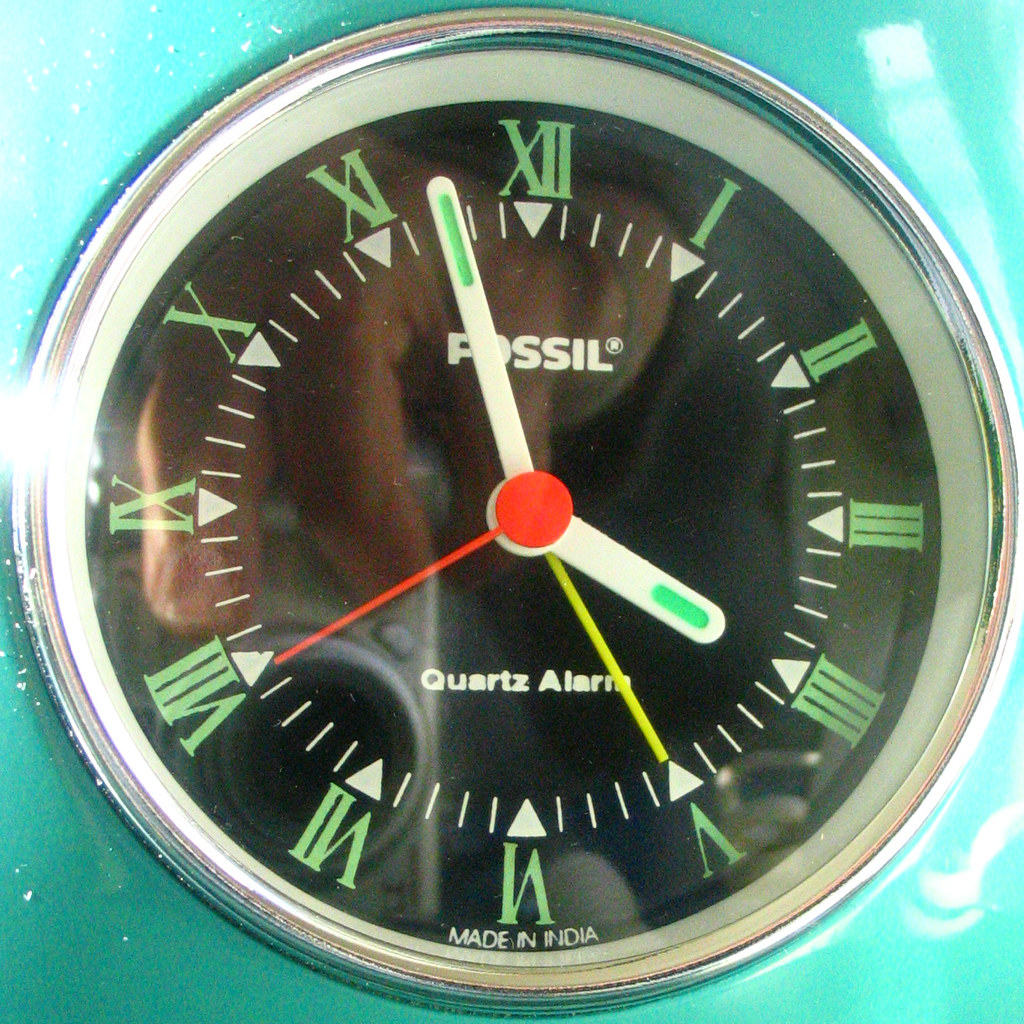This image showcases a black-faced Fossil watch with mint green Roman numerals and various intricate details. Prominently displayed on the watch face are the Fossil logo, a registered trademark symbol (®), the words "Quartz Alarm," and "Made in India" at the bottom. The numerals, along with some upside-down triangles as hour markers and hashtags marking each minute, are depicted in a mint green hue. The hands of the watch, featuring mint green indents, are primarily white, with a small rod in red and another in yellow, indicating seconds. The watch face is encased in a disc with a silver rim, set against a teal background, which might belong to the watch casement or band. An intriguing aspect of this photograph is the clear reflection on the watch's glass surface, showing a Caucasian man's hand holding a silver digital camera to take the picture.